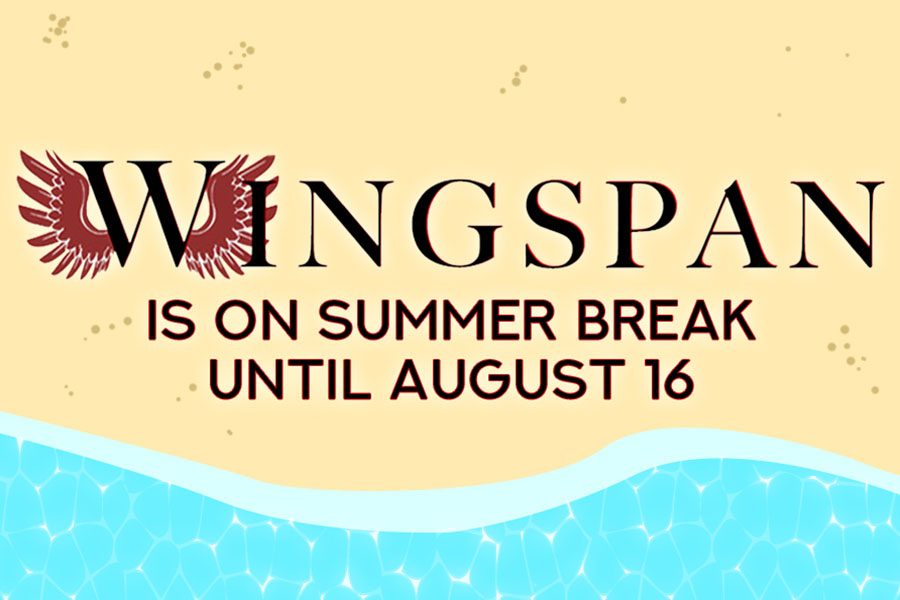The image is a horizontal rectangular advertisement designed with a modern illustrative beach theme. At the top, "WINGSPAN" is written in large, bold, uppercase serif font with purple wings adorning the W. Directly beneath in smaller, bold, uppercase sans-serif font, the text announces, "IS ON SUMMER BREAK UNTIL AUGUST 16TH." The background transitions from a pale peach or tan color at the top, resembling sand, down to a wavy light blue line that demarcates the surface of the ocean. Below this line, the bottom section is filled with a darker teal color, featuring a pebbled white texture, evoking the appearance of waves breaking onto the shore. The entire scene gives the impression of looking down at a beach coastline.